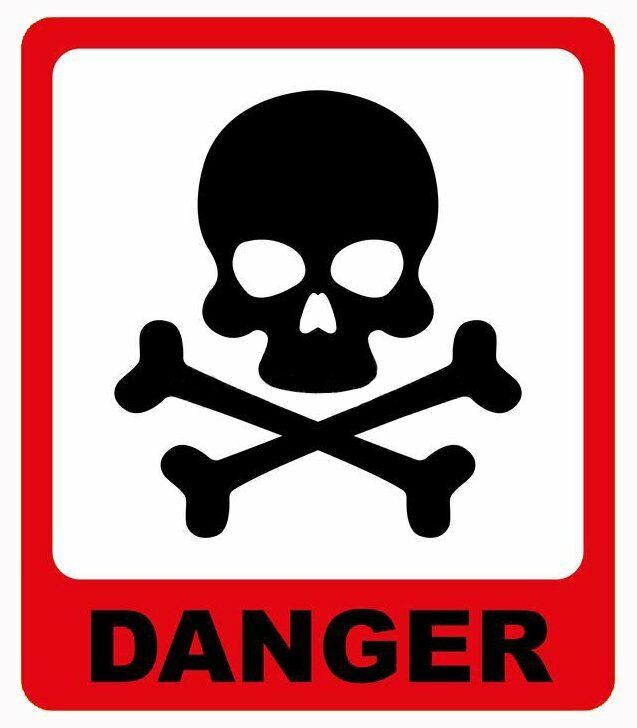The image depicts a classic danger sign characterized by its prominent red background and central white square. The white square is slightly rectangular and contains a black skull and crossbones symbol, which takes up most of the sign. This skull, rendered in a somewhat caricatured style with defined cheekbones, eye holes, and a nose cavity, denotes danger through its traditional imagery. Beneath the white square, the word "DANGER" is written in large, black block capitals against the red background. The stark contrast of colors—black on white for the skull and crossbones, and black on red for the warning text—ensures high visibility and makes the sign hard to miss. The overall design is straightforward, serving as an unequivocal warning marker.